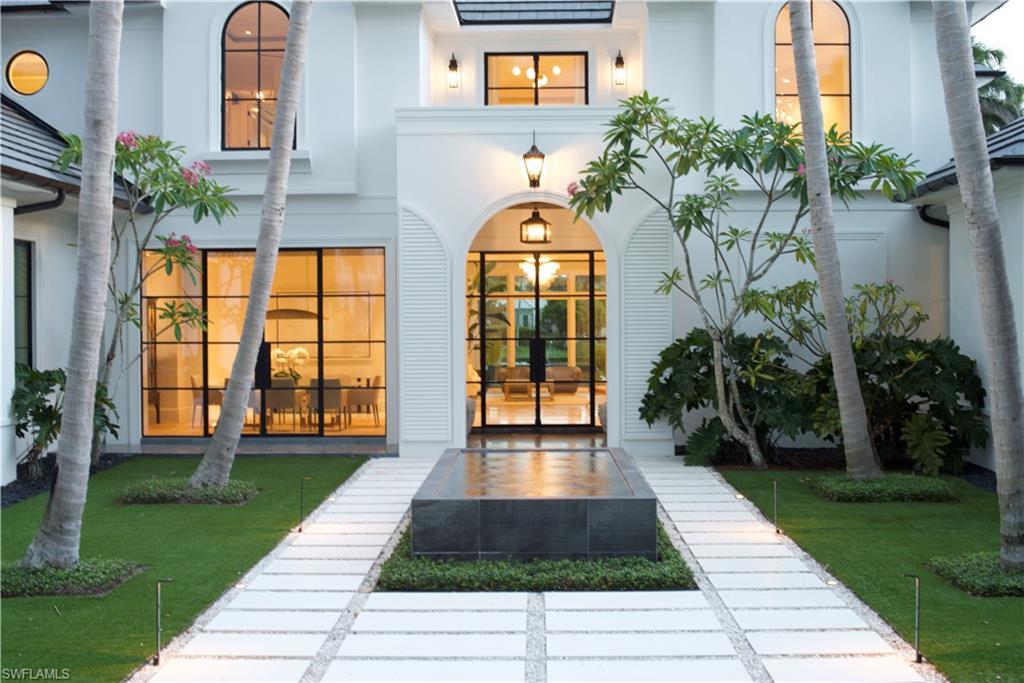This color photo captures an elegant courtyard in front of a white mansion or hotel. The building features large, black-divided glass windows and a central glass door with a rounded frame, allowing glimpses of warm orange lighting inside that illuminates furniture like a dining table and chairs. Outside, a white pathway leads to the entrance, flanked by well-manicured green grass and tropical trees with pink flowers. The trees have tall, grayish trunks resembling palm trees. Central to the courtyard is a rectangular, dark marble fountain or decorative bench, set amid a gray stone pebble ground and bordered by white paver tiles. Various plants adorn the house's base, complementing the overall serene and inviting atmosphere.